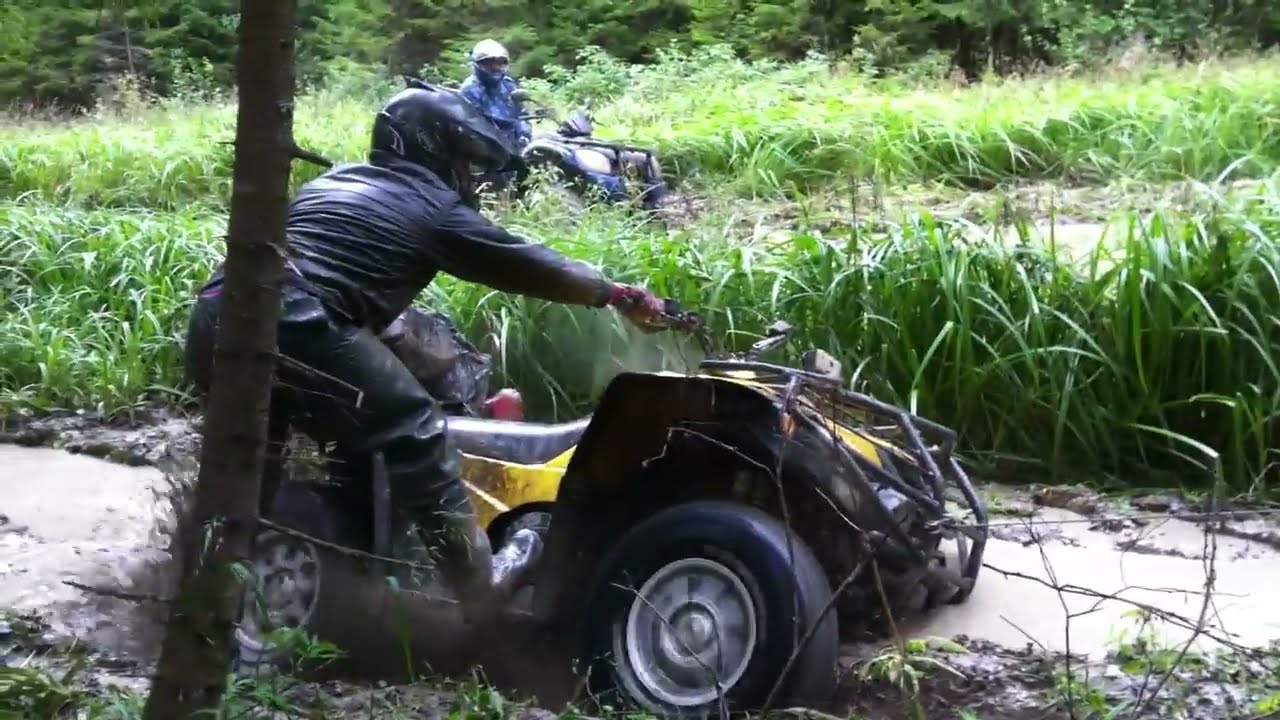In this horizontally aligned rectangular image, two people with ATVs are depicted navigating a dense, lush green area with waist-high grass. The person on the left is wearing a leather jacket, pants, and a black helmet, struggling to pull their yellow and black four-wheeler out of a large mud puddle, indicating they are quite wet. On the upper right part of the image, another individual wearing a white helmet is seated on a blue ATV, looking towards the person stuck in the mud. The setting is clearly outdoors, with tall trees featuring green leaves in the background, suggesting a dense, jungle-like environment. Additionally, there's a tree branch extending diagonally across the image, contributing to the overall rugged natural scenery. The ground transitions from dry dirt on the left side to the muddy water where the first ATV is stuck, further emphasizing the challenging terrain. The scene appears to be taking place in the middle of the day, illuminated by natural light.